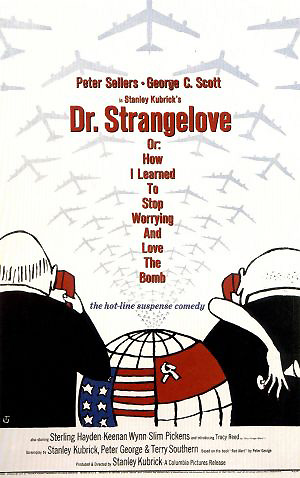This detailed movie poster features a white background with a large formation of gray bomber silhouettes at the top. Prominently displayed in bold red letters are the names "Peter Sellers" and "George C. Scott," separated by a dot. Below these names, in smaller red text, it reads "Stanley Kubrick's," followed by the larger title "Dr. Strangelove or: How I Learned to Stop Worrying and Love the Bomb." As a tagline, it includes "A Satirical Suspense Comedy." 

The lower section of the poster showcases cartoon drawings of two bald, slightly overweight men seen from behind. Each man holds a red phone to his ear. Positioned between them is a globe displaying flags of the United States and the Soviet Union. At the bottom of the poster, film credits appear in fine print, listing names such as Sterling Hayden, Keenan Wynn, Slim Pickens, and reiterating Stanley Kubrick's involvement. The artwork and text are indicative of the film's satirical tone and Cold War setting.